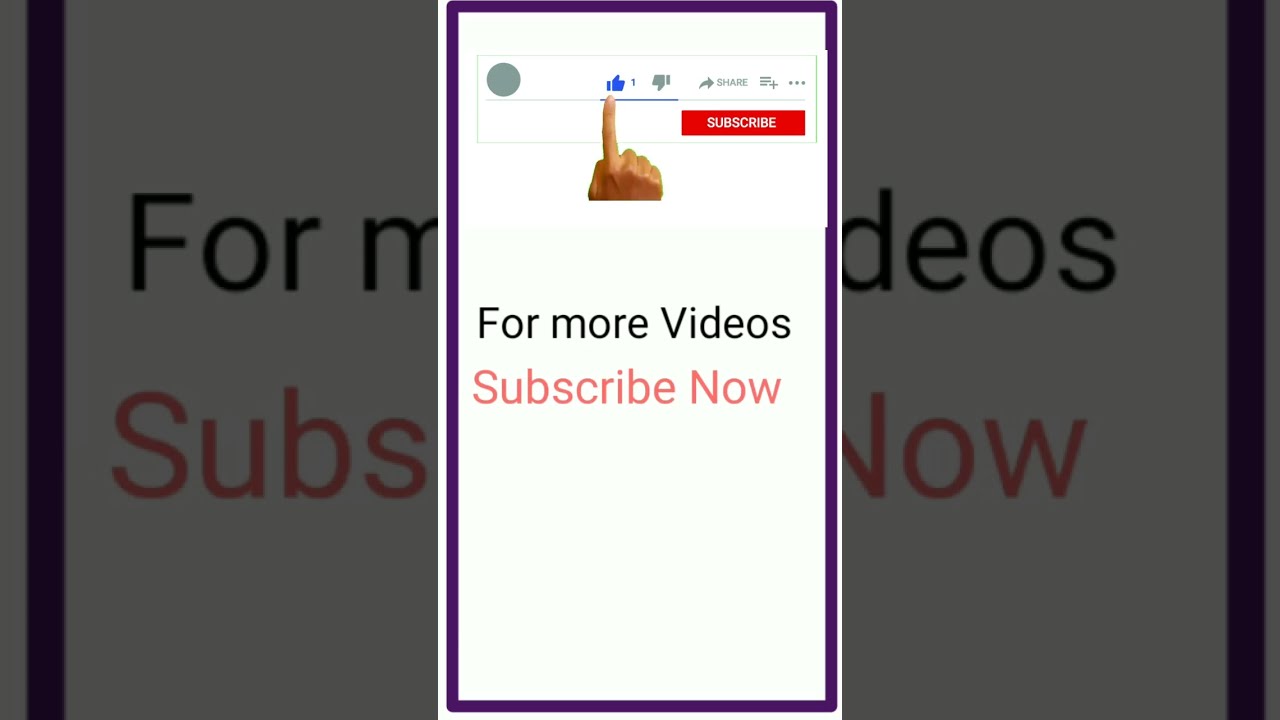The image is a composite of two layers on a screen, similar to a YouTube video interface. The background layer is a faded, grayish rectangle that spans the center, bordered on the left and right by blue bars. This background features the text "4 more videos" in black and "subscribe now" in red. Overlaying this is a prominent white rectangle with a dark purple border in the foreground. The same text, "4 more videos" and "subscribe now," is repeated in the center of this white rectangle, maintaining the same color scheme. At the top of the foreground layer, a disembodied hand points to a blue thumbs-up icon with a "1" next to it, indicating a like. Directly beneath it is a grayed-out thumbs-down icon. To the right of these icons is a gray arrow labeled "share," and below that is a red "subscribe" button with white text. The hand extending from the top stops at the wrist, and beneath it, the instructional text "for more videos" in black and "subscribe now" in light red is repeated.